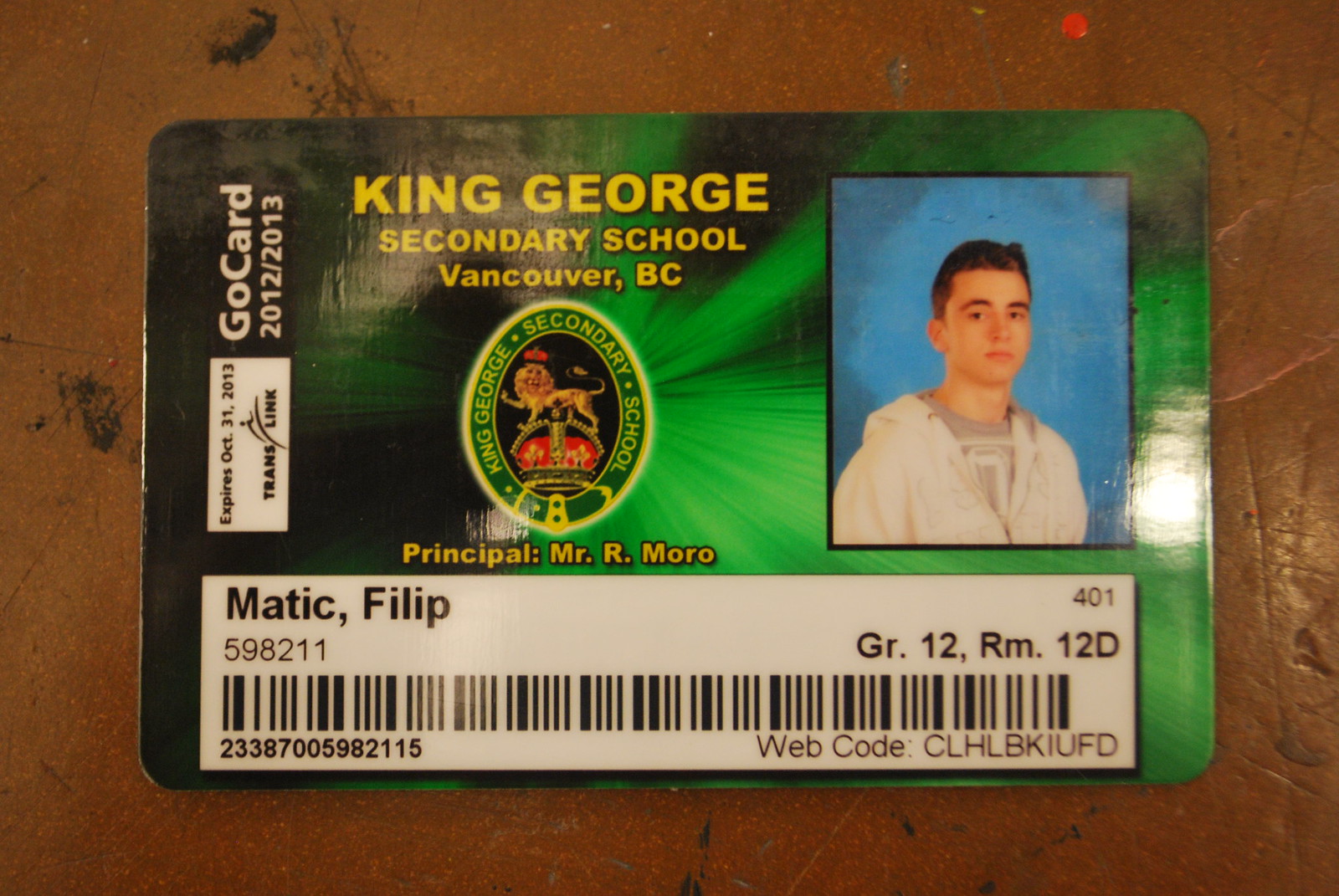The photograph captures a student ID card placed on a brown table, showcasing its detailed design and information. The ID card features a green background with splashes of black and rays of lighter green. On the right side of the card, there is a photograph of a young male student set against a blue backdrop. The student, dressed in a white hoodie over a gray and white t-shirt, is identified as Mateek Philip. 

Centrally positioned in bold yellow letters is the text "King George Secondary School, Vancouver, BC," accompanied by the school's logo—a lion atop a crown—below which reads "Principal Mr. R. Morrow." The left side of the card states "Expires October 31, 2013" and "Go Card 2012/2013." Below these details is a barcode with the number MATIC-FILIP-59821 and the web code CLHLBKIUFD. Additional information indicates that Mateek is in grade 12, room 12D. This ID card appears to be essential for accessing certain areas within the school.